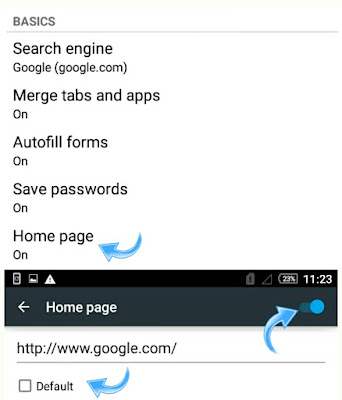The image is a detailed screenshot featuring a white background with various text elements and a few graphic components. 

At the top left corner of the image, the word "Basics" is prominently displayed with a thin gray horizontal line directly beneath it. Below this heading, there is a list of settings in black text, each followed by a status indicator in parentheses. The settings include:

- Search Engine: Google (google.com)
- Merge Tabs and Apps: On
- Autofill Forms: On
- Save Passwords: On
- Home Page: On

Approximately three-quarters down from the top, there is a gray strip with a black address bar. This strip contains small icons positioned at the left end. On the right end of the black strip above the gray bar, the battery icon indicates a charge of 23%, and the current time is displayed as 11:23.

Just below the gray strip, a section features white text that reads "Home Page," accompanied by a right-pointing arrow. Adjacent to this text is a blue slider, which is positioned towards the right-hand side. 

Three curved arrows are overlaid on various elements in the image for emphasis. The first arrow points to the "Home Page" text. The second arrow highlights the blue slider. The third, located below the others, points to a URL, "http://www.google.com." Underneath this URL is another thin gray line.

Finally, a checkbox labeled "Default" is found below the URL, with the third arrow specifically pointing at the word "Default."

This image showcases the configuration settings of a web browser in a structured and detailed manner.